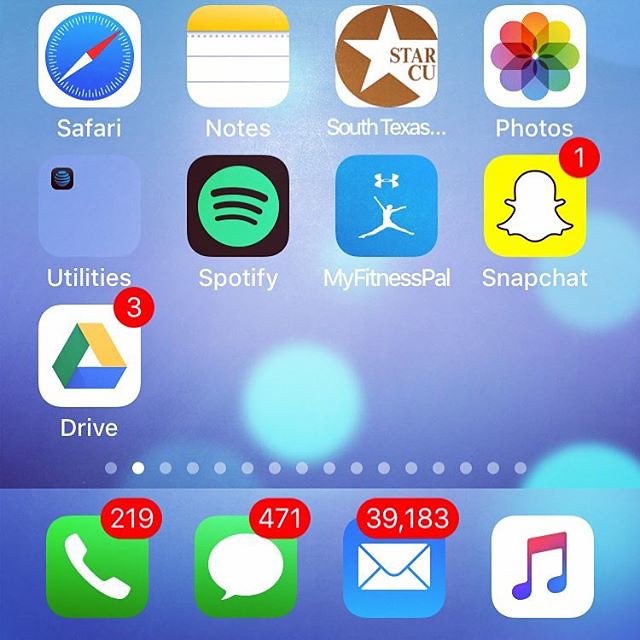The image displays a cropped view of an Apple screen, potentially from either an iPhone or an iPad, as indicated by the icons and layout, but lacks identifiable context clues such as the time, battery status, or Wi-Fi/cellular signal strength. The visible section reveals three rows of app icons:

1. **First Row:**
   - **Safari:** A web browser icon depicted as a compass with red and white markings on a blue background.
   - **Notes:** A white piece of paper with dotted perforations, resembling a notepad with a yellow header.
   - **South Texas (truncated):** A partially visible app, identifiable by a white star within a brown circle, labeled "star see you."

2. **Second Row:**
   - **Photos:** An icon resembling a multicolored circular flower with a central gray section that might appear as a loading symbol.
   - **Utilities Folder:** Inside, the AT&T app is represented by a black square with a blue-lined globe.
   - **Spotify:** A black square featuring a green circle with black radiating lines reminiscent of music or Wi-Fi signals.
   - **MyFitnessPal:** Characterized by a blue and white depiction of a gender-neutral person seemingly jumping.

3. **Third Row:**
   - **Snapchat:** Displaying a white ghost on a yellow background with one notification.
   - **Google Drive:** Represented by a multi-colored (green, yellow, and blue) trilateral shape that resembles a folded piece of paper, bearing three notifications.

At the bottom of the screen, frequent apps are docked:
   - **Phone:** A green icon with a white handset, indicating 219 missed calls or voicemails.
   - **Messages:** Green with a white speech bubble, showing an extensive 471 unread messages.
   - **Mail:** A blue icon with a white envelope, reflecting a staggering 39,183 unread emails.
   - **iTunes (Older Version):** A white icon with intertwined music notes.

Additionally, the numerous screen dots at the bottom suggest the user has over 15 different screens filled with icons, indicating an exceedingly busy and possibly disorganized digital life.